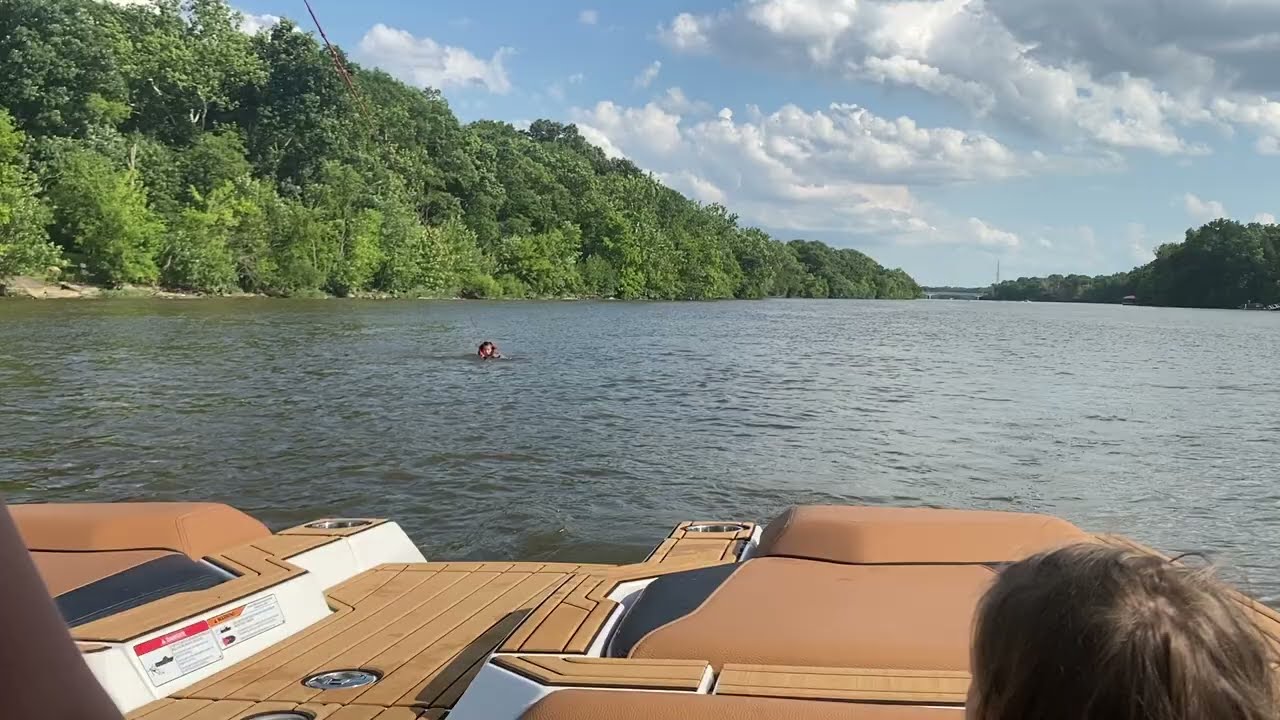In this detailed outdoor photograph, we observe a beige and white speedboat, momentarily stationary on a wide, greenish-brown river under a sunny and slightly cloudy sky. Only the back portion of the boat is visible, revealing cup holders, possibly a cooler handle, and some of the engine. In the lower right of the image, we can see the back of someone's head with light brown hair, facing away from us. In the water behind the boat, a girl prepared for water skiing is partially submerged, with just her head above the water and a ski line connecting her to the boat. The riverbanks on both sides are densely lined with trees, with traces of a sandy beach peeking through near the water's edge. The backdrop features a beautiful blue sky dotted with scattered, fluffy white clouds, creating a picturesque and serene scene.